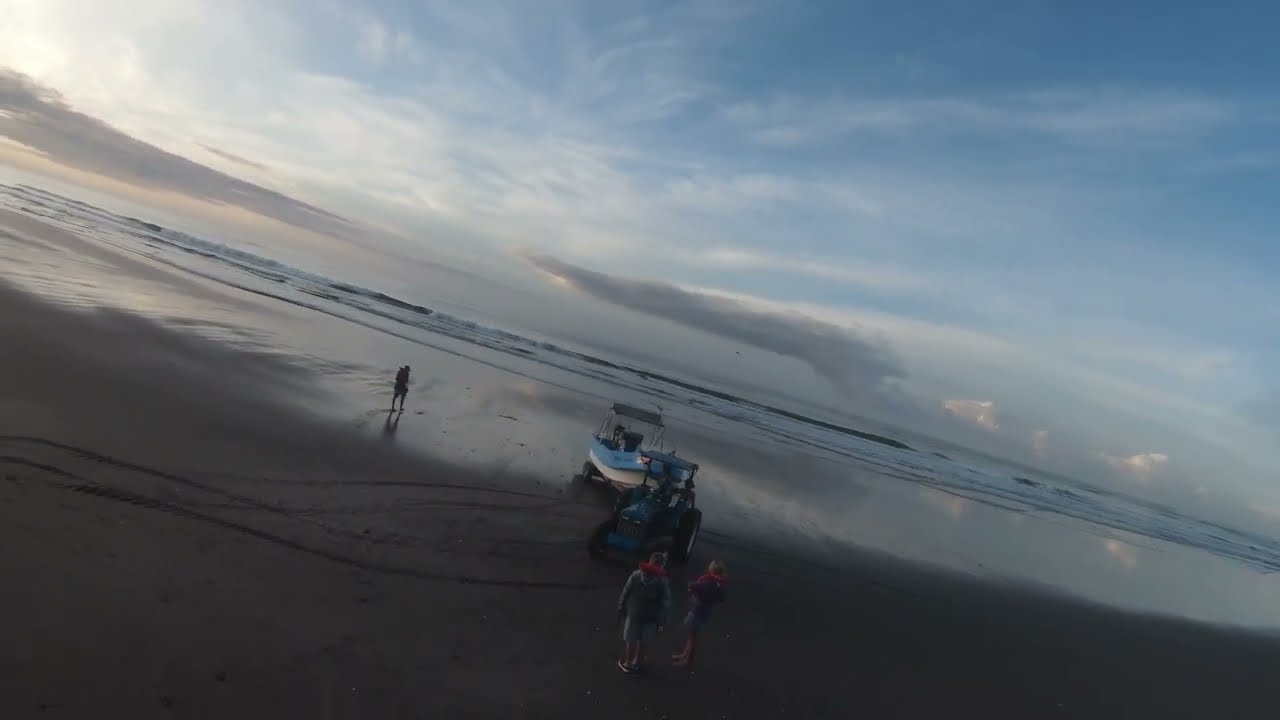This photograph captures a serene shoreline scene, taken at an angle where the beach descends from the top left to the bottom right. It's either early morning or late evening, enveloped in a dim light that accentuates the moody atmosphere. The focal point is a blue tractor pulling a white and blue boat on a trailer out of the water, with three people accompanying it—two in the middle of the frame, a man and a woman observing the process, and a third person walking along the water's edge. The beach itself transitions from a dry section of gray sand to a glossy wet sand nearer to the ocean. Waves gently crash onto the shore, their movements mirrored on the wet sand. Above, the sky is a tapestry of clouds—from darker ones near the horizon to lighter, wispy formations higher up—creating a layered effect. Tire tracks from the tractor and trailer add a rustic touch to the expansive sandy beach stretching into the background.